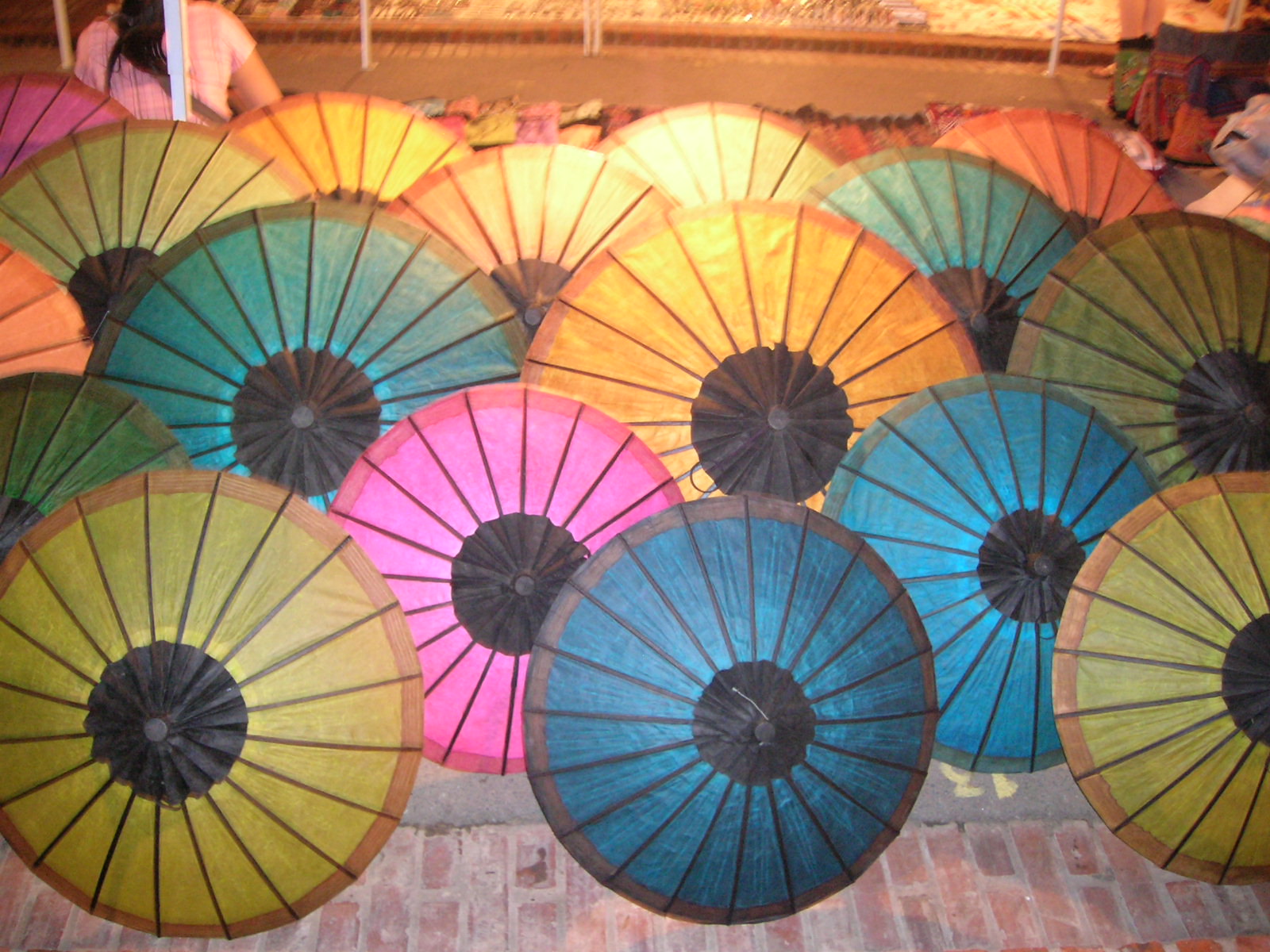This photograph captures a vibrant display of approximately 25 colorful paper parasols, arrayed on a red brick floor. The parasols, showcasing hues of blue, pink, yellow, and green, each feature dark ribs and borders in varying shades of brown, pink, and orange. The translucent paper allows light to shine through, accentuating their vivid colors. They are meticulously arranged in rows, with larger and smaller parasols interspersed, giving the impression of a market stall.

In the foreground, there's a distinct pattern: three yellow, blue, and yellow parasols in the front row, followed by green, pink, and blue in the next, then blue, yellow, and green with hints of an orange parasol on the left. Further back, the arrangement continues with green, yellow, and blue, and towards the rear, partially out of frame, are pink, yellow, yellow, and orange parasols. Additional colorful items are visible behind them.

In the background, a woman with black hair in a ponytail, dressed in a pink t-shirt and carrying a bag, faces away from the camera. Another pair of legs, visible from below the knee, also appears. The setting suggests a market or vibrant street scene, with fabric bags scattered in the background, enhancing the bustling atmosphere. The brick pavement is framed by brick curbs, hinting at a walkway bordering a garden area.